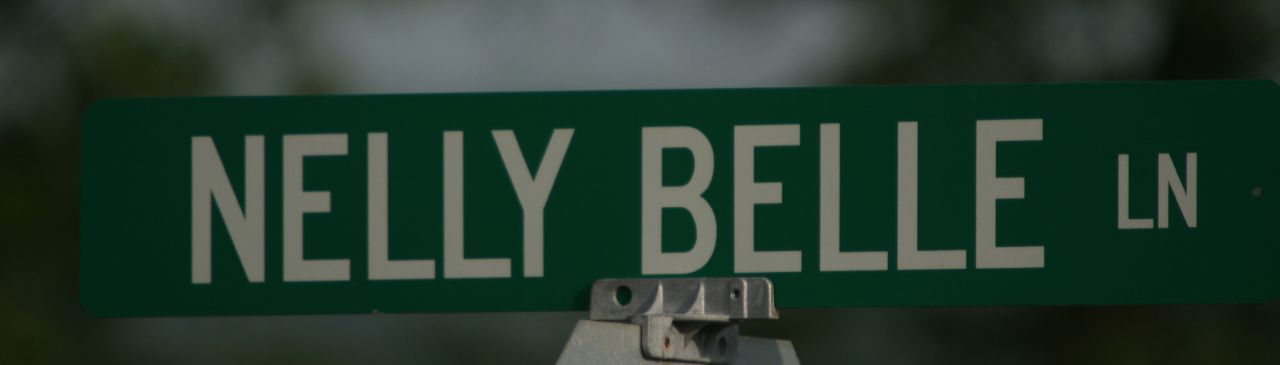The photograph is a long, narrow horizontal image taken outdoors of a street sign during dark lighting conditions. The sign, which is predominantly centered in the frame, is green with white capital letters that read "NELLIE BELLE" and in smaller font to the right, "L-N." The sign appears to be in pristine condition, with no visible damage. It is mounted on top of a pole using a gray cast metal bracket. The background is mostly dark, with a slightly lighter spot in the upper left portion, and is very blurred, providing no distinguishable features except a hint of gray sky and possibly some foliage. The image focuses on the street sign, which fills most of the frame, and reveals a clear though dimly lit representation of "NELLIE BELLE LANE."